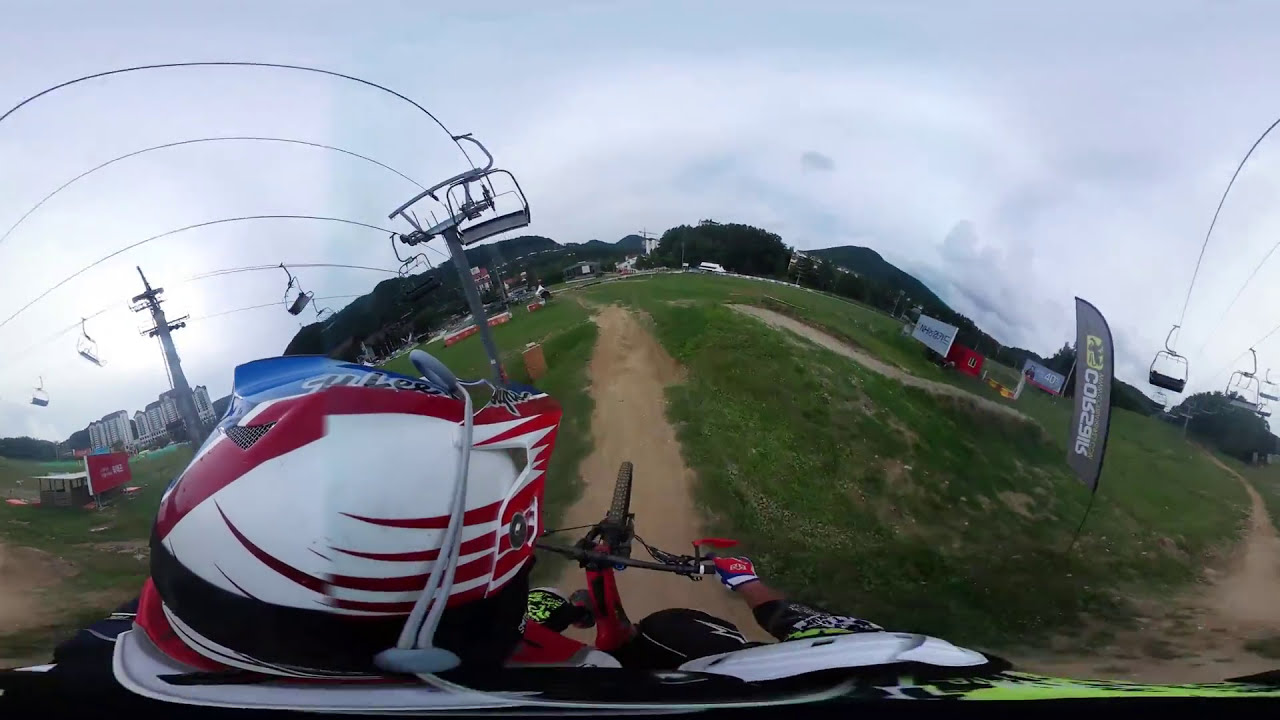In this detailed and dynamic image, we see an overhead view of a person riding a red mountain bike on a dirt track, flanked by grass on both sides. The photograph appears to be taken with a 360-degree camera, possibly a GoPro, which causes some distortion: the helmet looks unusually large, the arm appears elongated, and the bike wheel seems small. The cyclist is wearing a red, white, and blue helmet, red gloves, and white and black padding, and is centered towards the bottom of the image. The scene is set outdoors, likely during the middle of an overcast day, as the sky is completely filled with gray clouds.

The rider is pedaling swiftly, possibly with the front wheel slightly off the ground, indicating dynamic motion. Overhead, we can see a ski lift running alongside the dirt trail, suggesting that this may be a ski slope repurposed for biking during the summer. In the background, there are various objects that hint at human activity, like signs, sponsors' banners, parking areas, high-rise buildings, and other structures. Farther off, mountains and trees are visible, contributing to the expansive and busy atmosphere of the scene. No text is readable within the image, further emphasizing the focus on the vibrant action and the rich details of the surrounding environment.